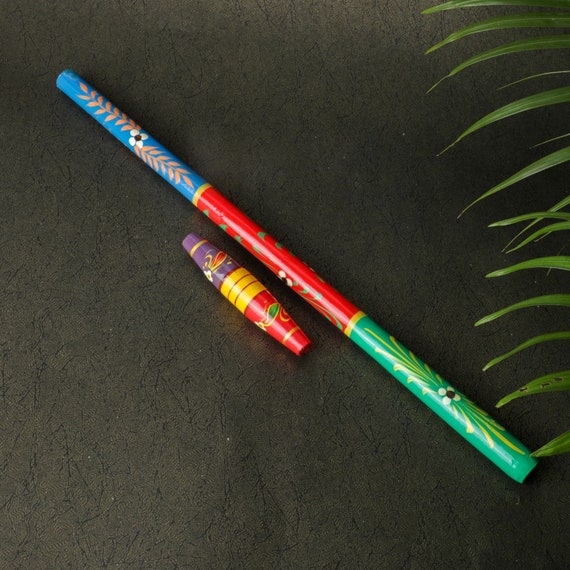The image depicts a colorful, intricately decorated toy, likely intended for children, positioned on a black surface. The main feature of the toy appears to be a stick that stretches diagonally from the upper left to the lower right of the frame. The stick is vividly adorned, starting with a blue section at the top that transitions into a red middle section and ends in a green segment, each part embellished with ornate floral designs. Notably, the blue section at the top features gold flowers. Adjacent to the main stick, there is a smaller, separate stick positioned nearby, about one-third the size of the main toy. This smaller stick is distinct with its purple left side, red right side, and three gold bands around a slightly wider center. Additionally, on the right side of the image, a plant is visible, contributing to the scene’s detailed composition. Despite its rich and ornate appearance, the cultural or national origin of the toy remains unclear.